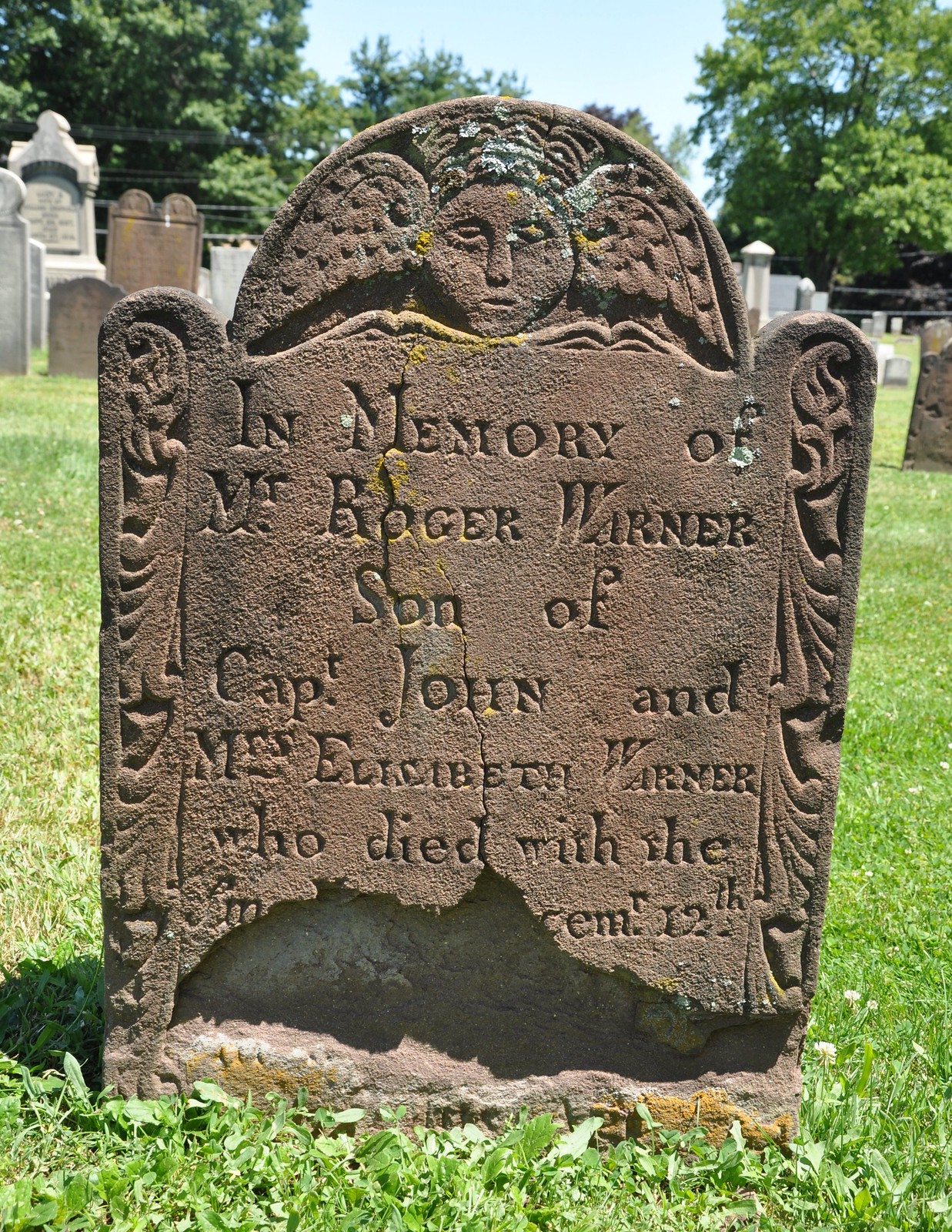In the image, there's an incredibly old and degraded tombstone standing amongst other headstones in a cemetery. The ground around it is covered in lush, green grass. The tombstone itself is made from a brown material, possibly brown stone or cement. At the top of the tombstone, there's an engraved circular human face with wings on either side, resembling an angel. Below this intricate engraving, the inscription reads: "In memory of Mr. Roger Warner, son of Captain John and Elizabeth Warner, who died with her..." Unfortunately, the lower part of the tombstone is broken and crumbling, making it impossible to read the rest of the text or determine the date of death. The overall condition of the tombstone suggests significant aging and decay.